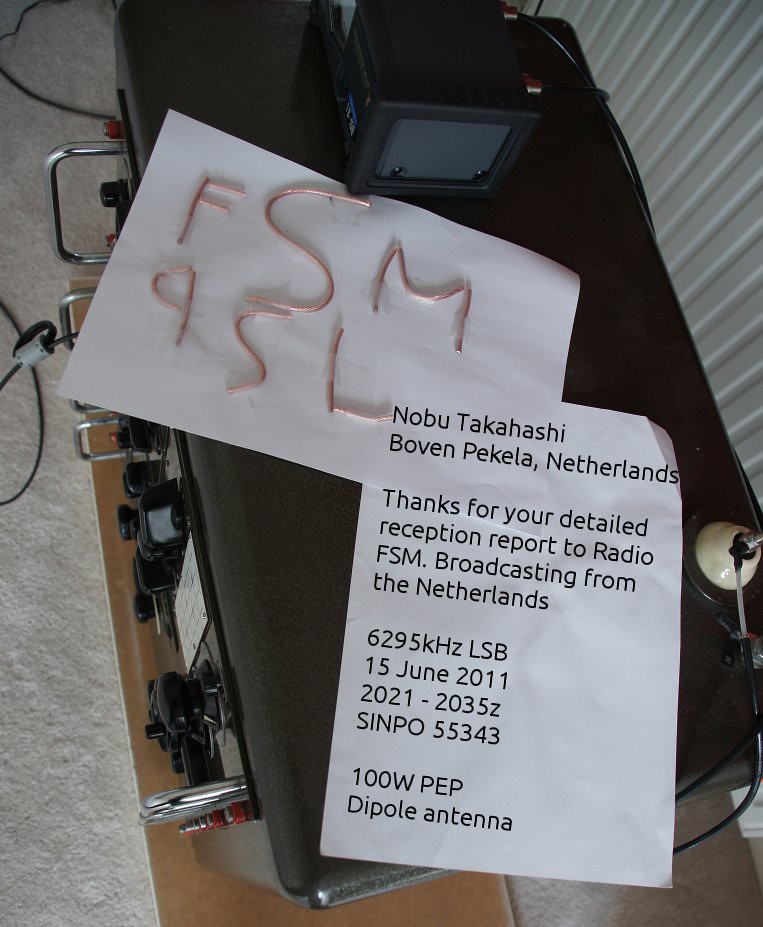The image shows a large rectangular electronic device, likely a radio, situated on a brown table with a black top, featuring several knobs and wires. Two pieces of paper rest on the top of the device. One piece of paper has the letters "FSM 9SL" formed out of copper wire. The other piece is a typewritten note that reads: "Nobu Takahashi, Boven Paquila, Common Netherlands. Thank you for your detailed reception report to Radio FSM, broadcasting from the Netherlands, 6295 kHz LSB, 15 June 2011, 2021 to 2035Z, SINPO 55343, 100W PEP dipole antenna."